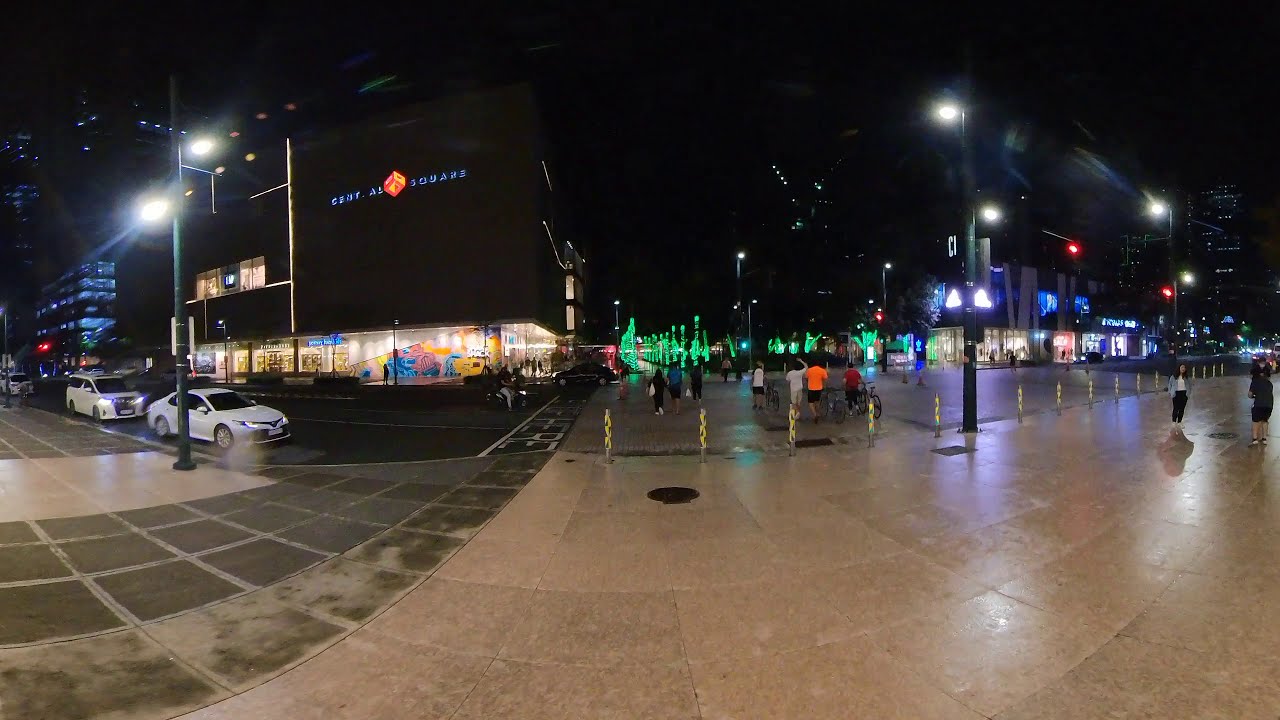The image captures a vibrant nighttime scene in a bustling city. Taken using a fisheye or wide-angle lens, the photograph showcases extensive street views on both sides. In the center, a large crosswalk is filled with pedestrians wearing orange, red, white, and blue shirts, heading towards a street adorned with green, illuminated decorations. The background reveals a mix of dark and lit-up skyscrapers, indicating a big city. Prominently, on the left side, a building with the logo "Scent Ale Square" is brightly lit, standing next to a recognizable Gap clothing store. Further left, larger buildings with blue-lit windows, possibly apartments, line the street. Several vehicles, including a white sedan and a white minivan, are seen pausing to let pedestrians cross. On the right side, more stores and shopping areas are visible, along with additional traffic lights and people standing around. The streets are also dotted with street lighting and some barricades for pedestrian safety. The sidewalk varies in color—tan and gray—and is sectioned off into segments.